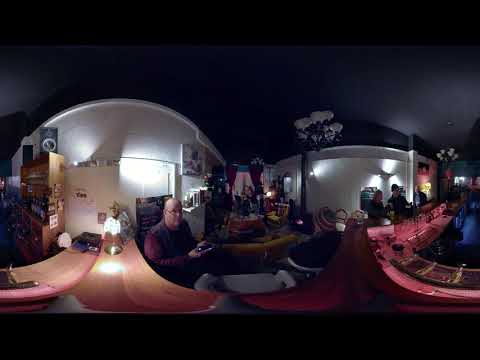The image is a highly distorted 360-degree, fisheye view of a pub or bar interior, making certain objects appear larger or smaller than they actually are. Central to the scene is a bald man wearing glasses, seated at the bar with his hands in front of him, looking upward. The bar itself, which is L-shaped, features red lighting underneath the serving area, contrasting with the darker black and blue hues of the walkway and flooring. The ceiling is dark with a mix of lighting, including chandeliers and smaller lights that add to the ambiance. To the left, there is a white wall and some cabinetry highlighted by the lighting, with what appears to be a wooden table nearby. On the right, several patrons are either seated or standing by the bar. A bartender, dressed in blue, stands behind the bar. The central area of the image features some sofas, couches, and seats, indicating a cozy lounging space amidst the skewed perspective.